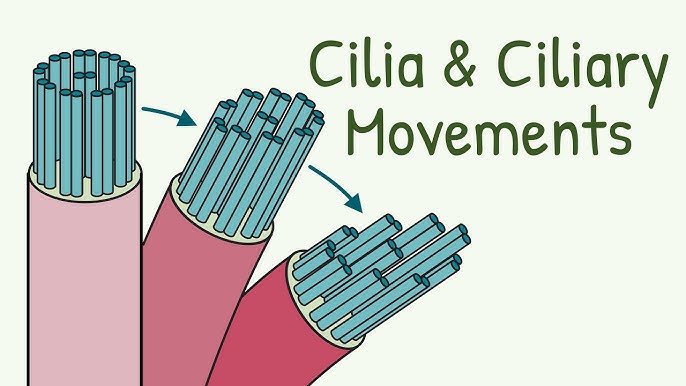This detailed anatomical illustration titled "Cilia and Ciliary Movements" features three progressively bent structures representing cilia within a light blue-gray background. The labels are in dark green text. Each cilium is encased in a colored outer coating: pink on the left, darker pink in the center, and reddish-pink on the right. The cilia are shown tilting more towards the horizontal as you move from left to right. Metal rod-like structures extend from their centers, indicating their internal composition. Blue arrows point from one cilium to the next, demonstrating the directional progression of movement. This educational piece likely illustrates the mechanism of ciliary motion, possibly within respiratory anatomy, highlighting how cilia bend and the resultant effects on their function.